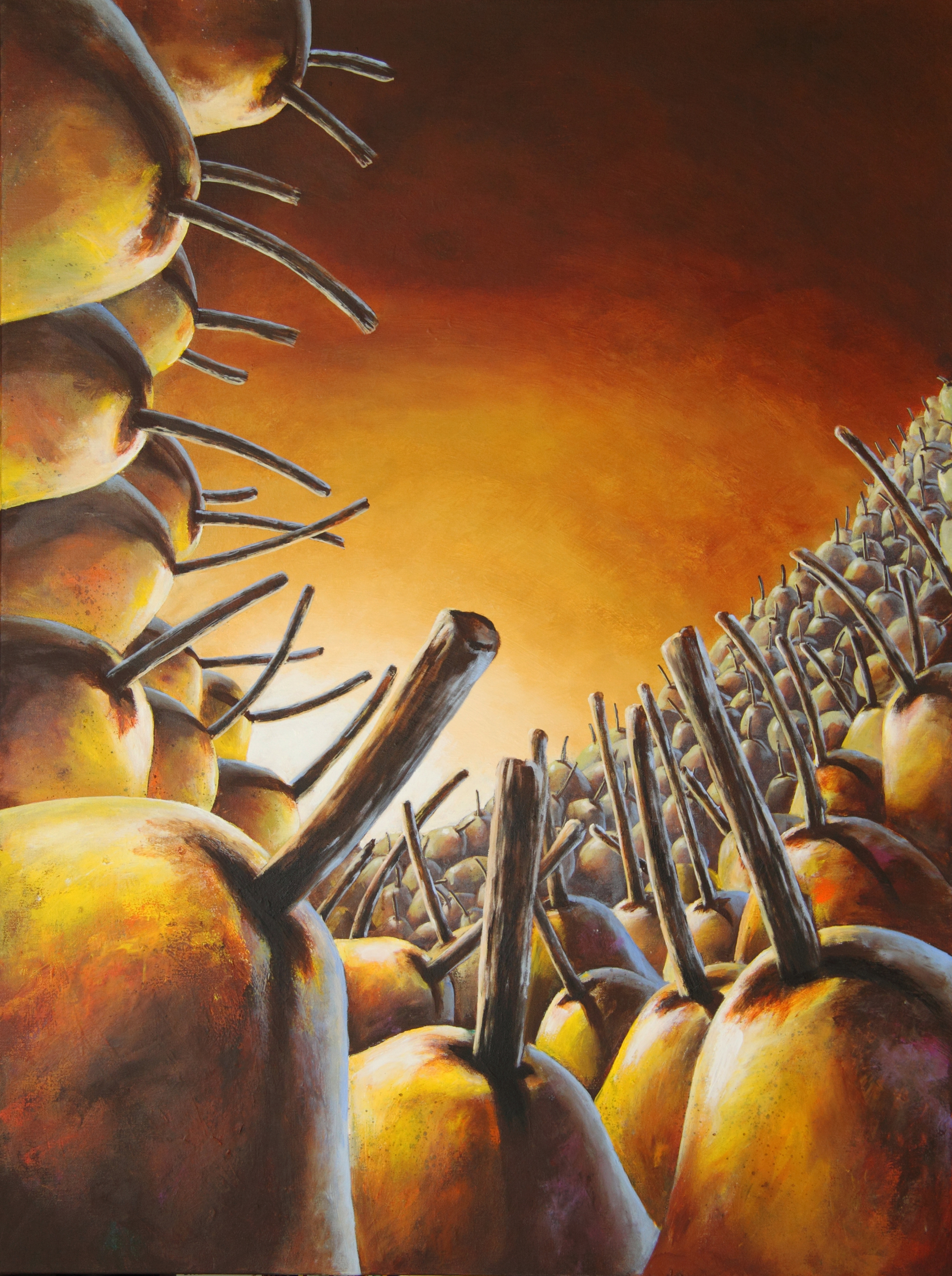This painting presents a vast, abstract landscape dominated by hundreds of pears, rendered in a palette of browns with subtle hints of green. These pears, each adorned with a prominent brown stem, fill what seems like a giant hole, creating the impression of a valley of pears. Viewed from an upward angle, the perspective suggests we are looking from the depths of this valley towards the sky. The sky itself transitions from dark brown at the top to lighter shades towards the center. The foreground features larger, more detailed pears, while those further away appear smaller. Interspersed amongst the pears are yellow, red, and black fruits, contributing to the abstract composition. Illuminated by a reddish light source from the center left of the image, the scene takes on a warm, almost otherworldly glow. The fruit arrangement slopes from the top right down to the bottom and up again to the top left, creating a dynamic flow within the image. Despite its complex arrangement and the absence of a visible signature, the image captures a surreal yet detailed representation of an abundant harvest under a twilight sky.